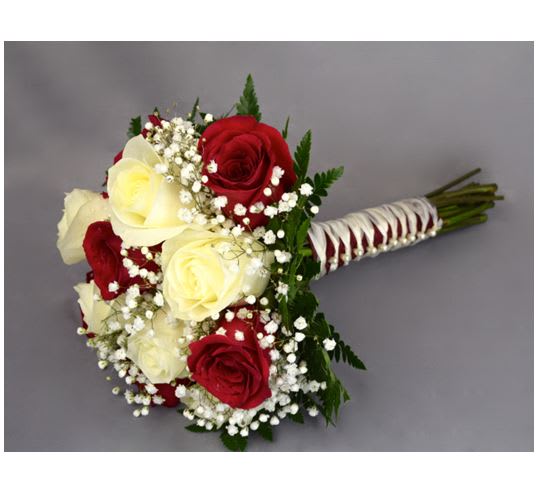The image captures a meticulously arranged bouquet of flowers, prominently featuring a mix of roses and delicate white flowers. The bouquet is composed of approximately ten roses, a blend of four to five red roses and five white roses, intricately bound together with an artistic arrangement of string that resembles the handle of a Japanese katana. The floral arrangement includes dozens of tiny white flowers akin to little daisies, interspersed among the roses, adding a delicate touch. Surrounding the roses are green leaves that enhance the bouquet's lush appearance. This artistic creation rests on a solid, softly varying gray surface, providing an understated but elegant backdrop that highlights the vibrant colors and intricate details of the bouquet.